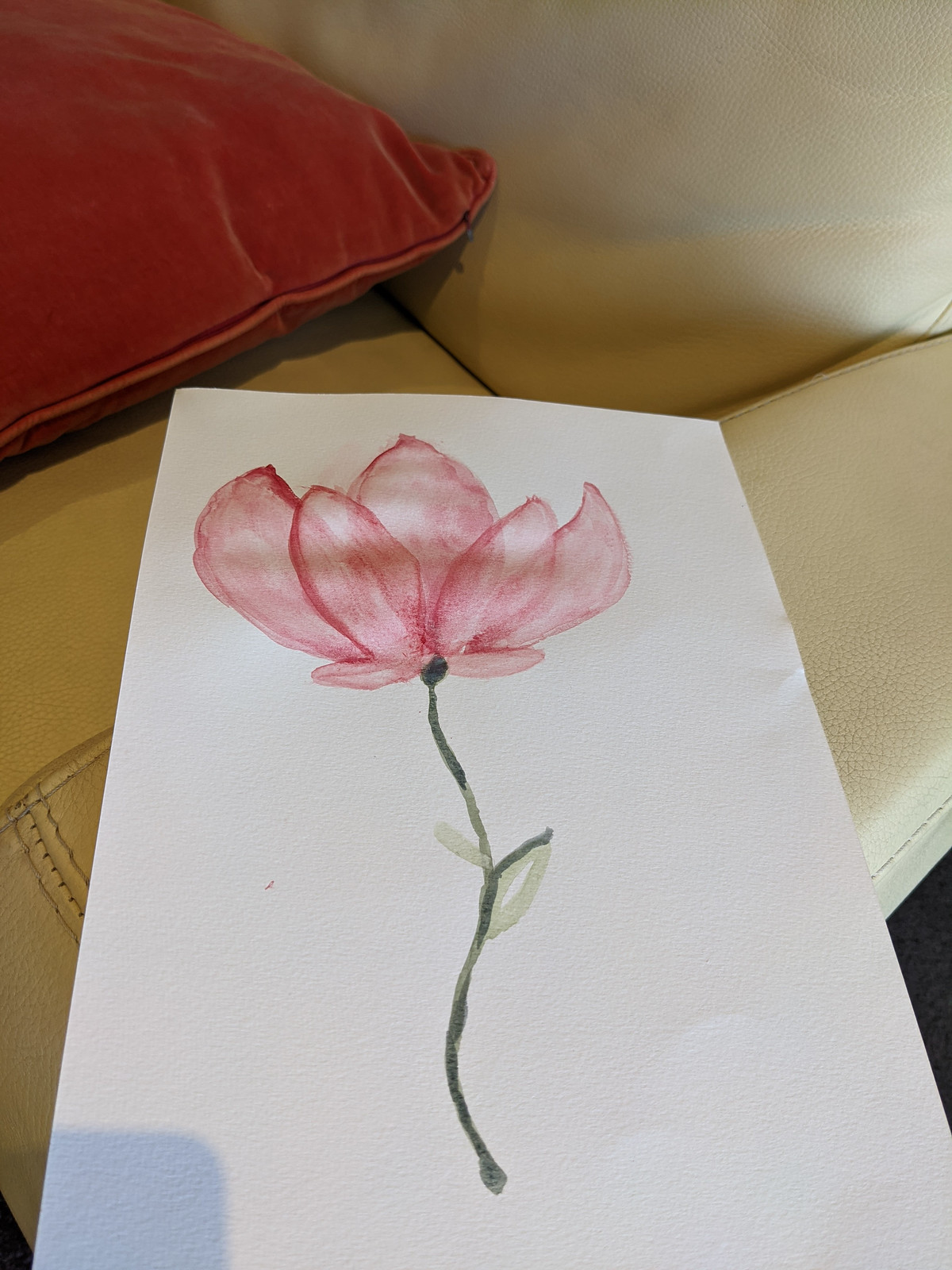The image is a vibrant, color photograph taken in a portrait orientation, showcasing an intricately hand-drawn illustration of a flower on a textured white piece of paper, which appears to be a special type of art paper due to its visible bumps and grain. The illustration is done in colored pencil, featuring a curved, undulating green stem that emerges from the bottom of the paper. On the right side of the stem, a large leaf extends outward, while on the left side, just above the larger leaf, a smaller leaf is positioned almost in a side profile. The attention-grabbing flower at the top has pink petals, artfully shaded with darker pink along the edges. The flower is depicted from a low-angle, side profile view, emphasizing its three-dimensional appearance.

The white paper rests on the thick arm of a cream-colored leather couch or armchair, which is detailed with white stitching. In the upper left corner of the photograph, a red cushion is partially visible, resting on the seat part of the chair, adding a pop of color to the setting. The overall composition combines the textured quality of the paper and the rich colors of the flower and surroundings, creating a visually engaging and detailed scene.